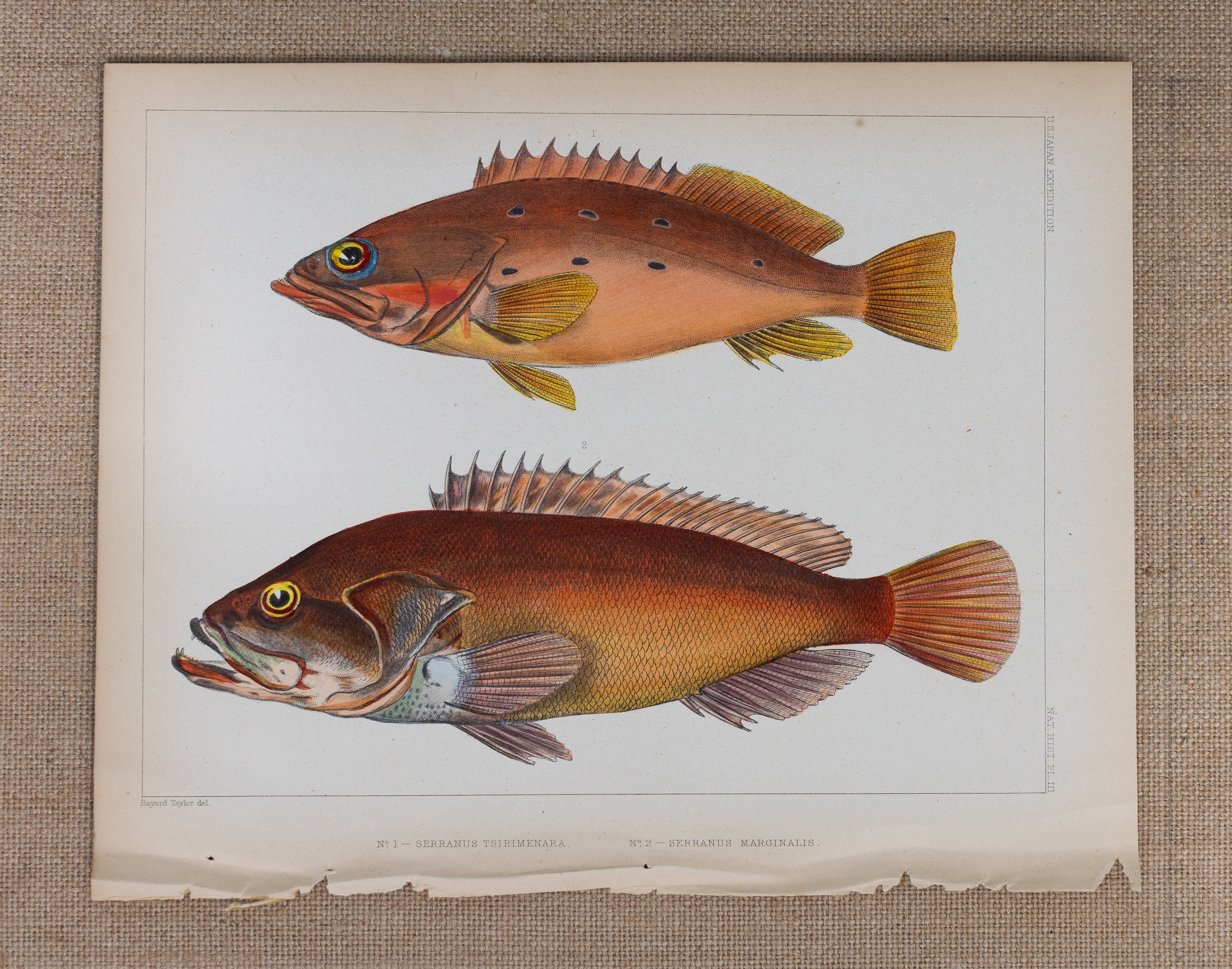This image depicts an old, tattered page, seemingly torn from a book or calendar, showcasing an illustration of two fish. The page itself is white or sun-faded white, with visible rips, bends, and a crinkled texture at the edges, indicating its age. It is placed on a plain, burlap-like fabric background. 

The fish, drawn horizontally one above the other with a small gap in between, exhibit a range of colors including brown, coppery yellow, red, tan, and pink, with some blue accents. The fish on the top features red markings, yellow fins, and a blue ring around its eye, while the fish on the bottom, larger in size, has more brown fins, a yellow eye, and an open mouth. Both fish have prominent spikes along their bodies.

The illustration is surrounded by a faint, light black rectangular outline, and there are barely legible names printed beneath each fish, along with some other fine, unreadable text around the line border. The two fish dominate the page, making it a detailed visual representation likely intended for educational or illustrative purposes.